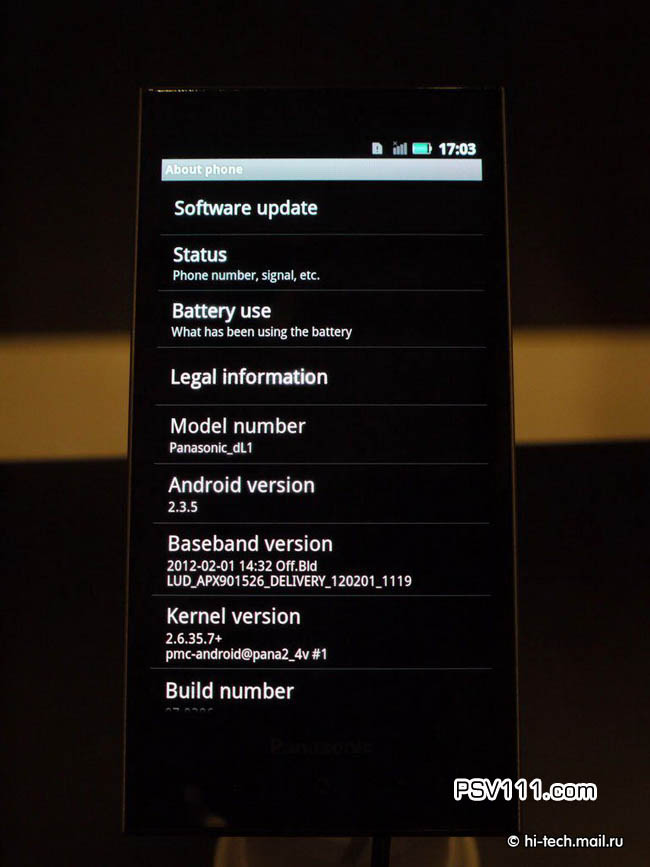This image depicts a single object, an Android phone, centrally positioned against a dark background that obscures any additional details in the room. The phone's screen is active, displaying the "About Phone" settings menu. At the top, the screen shows the battery level, volume level, and the time. Directly beneath, in a blue banner, it says "About Phone." Below this banner, the menu lists various informational categories including Software Update, Status (with details like phone number and signal), Battery Use, Legal Information, Model Number (Panasonic DL1), Android Version (2.3.5), Baseband Version, Kernel Version, and Build Number. At the bottom of the image, distinct from the phone screen, URLs "psv111.com" and "hightechmail.ru" are visible. The visible colors on the phone include black, white, gray, green, and light brown, with an indistinguishable background that features a brown and beige gradient, potentially indicating a store display setting.